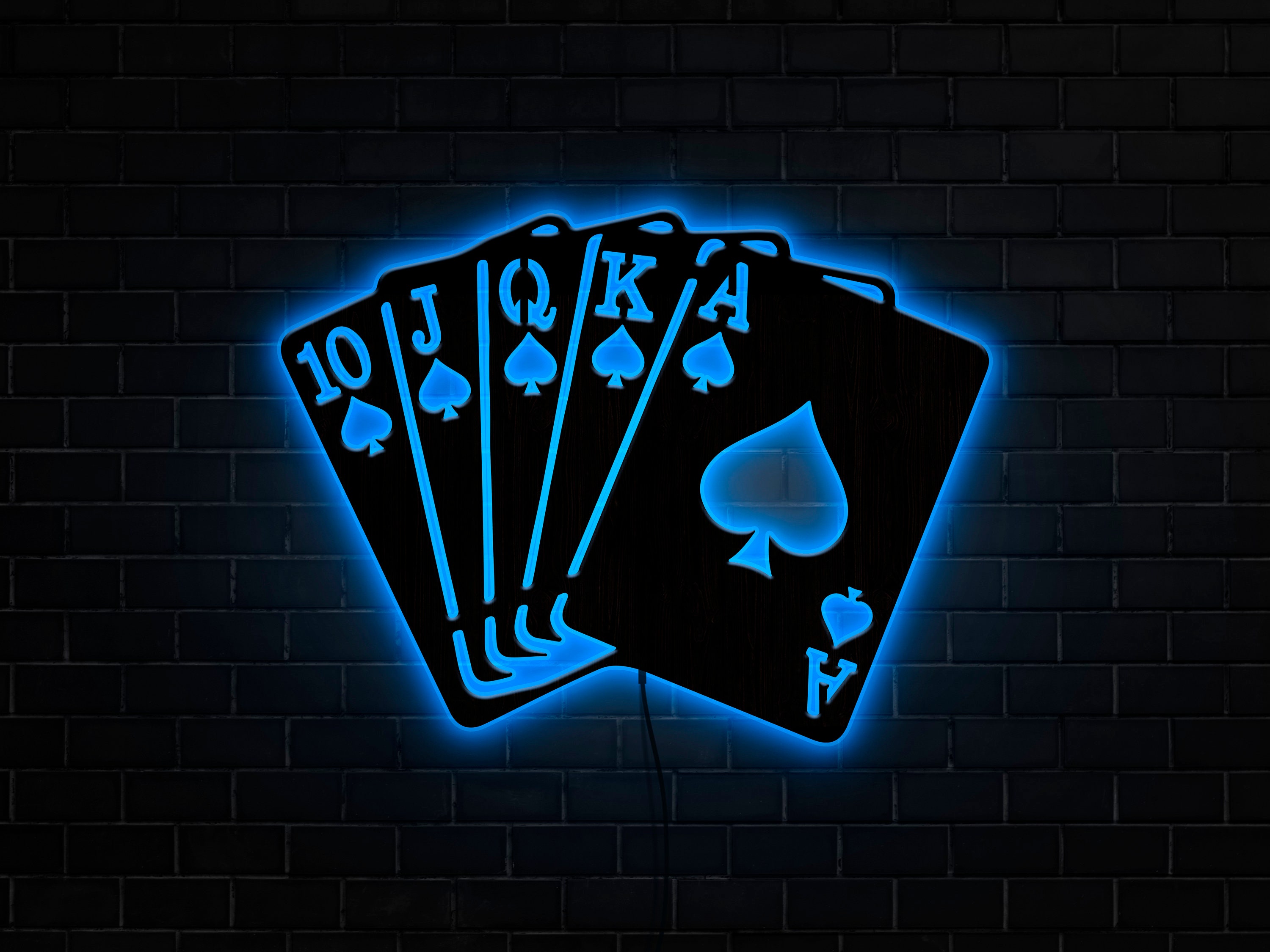This visually striking image captures a color photograph of a unique neon light display set against a black brick wall. The central feature is a luminous representation of a hand of cards from poker, specifically the 10, Jack, Queen, King, and Ace of Spades, arranged from left to right with the cards overlapping and the Ace of Spades on the far right being the most prominent. The cards themselves are black, and their numbers and suits are intricately cut out, allowing the blue neon light to glow through the edges and cut-out sections, creating an ethereal effect. A visible black cable runs downward from the base of the display. The neon light, which is backlit, casts a subtle aura onto the brick wall, emphasizing the design details and contributing to the nightclub-like ambiance of the scene.